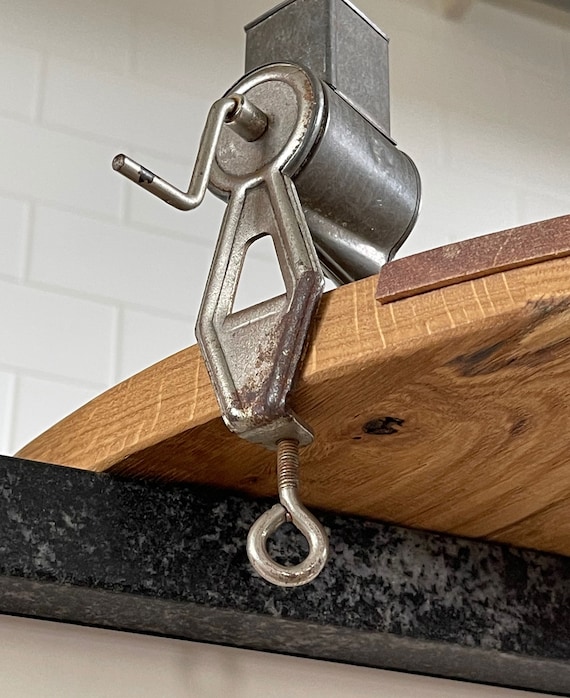The close-up image depicts a silver, antique-looking cylindrical apparatus attached to the underside of a thick wooden surface, which appears to be part of a desk or countertop. The apparatus is mounted by a slightly rusty screw. The contraption features a crank handle, suggesting it is operated manually, and it extends to an open square top. It's ambiguous whether the device is an old-fashioned pencil sharpener, a pasta maker, or a meat grinder. The backdrop reveals a white tiled wall, and the wood is seated on what seems to be a black marble or stone surface. The viewpoint from below makes the apparatus appear larger and highlights the intricate details of its construction, leaving its exact function somewhat unclear.